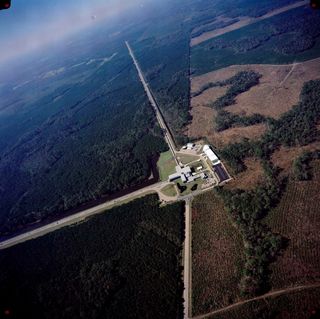This high-altitude, aerial photograph, seemingly taken from an airplane, captures a remote, flat expanse of land. At the center, three roads converge into a clearing containing what appear to be large industrial buildings, potentially a manufacturing plant or warehouse. These buildings are primarily long and white, set amidst a blend of grass fields and parking areas. The clearing, which resembles a square cutout, is surrounded by dense forests on the left and a mix of sparser woods and brown grassy areas to the right, possibly agricultural land. The left corner of the image hints at the horizon, contributing to an impression of vastness, though the sky above appears dark gray fading into a lighter gray. The scene, likely taken during daytime but under diffuse lighting, offers a stark contrast between the green, densely wooded left section and the more varied right section, showcasing the region's diverse landscape elements.